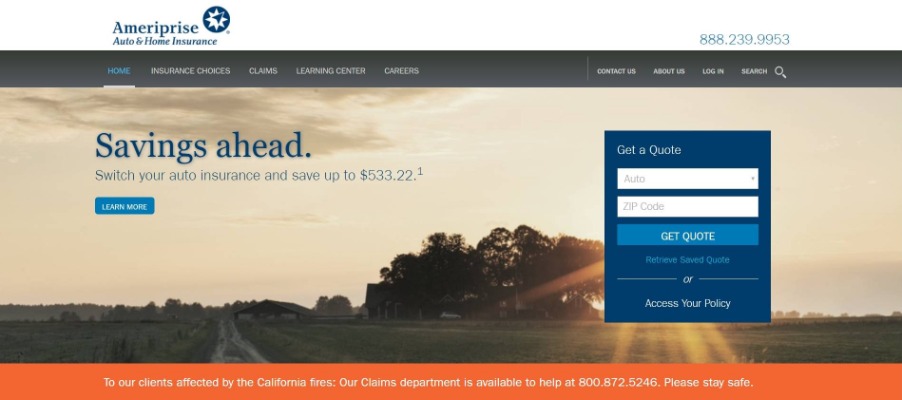The screenshot depicts the AmeriPrize website homepage, designed for their Auto and Home Insurance services. 

In the top-left corner, the AmeriPrize logo is prominently displayed alongside the company name. Beneath this, the text "Auto and Home Insurance" is clearly visible. Opposite in the top-right corner, the AmeriPrize phone number is provided for immediate contact.

Directly below this header section is a dark horizontal navigation bar with several clickable tabs. The Home tab is underlined, indicating that it is the current page. Other tabs include Insurance Choices, Claims, Learning Center, and Careers. Additionally, on the far right of the navigation bar are options for Contact Us, About Us, Login, and Search.

The main body of the page features a full-width background image depicting a picturesque rural landscape. This image includes a dense forest on the right, expansive farmland on the left, and an open sky with scattered clouds overhead.

Overlaying this background image in bold, white text is the headline "Savings Ahead. Switch your auto insurance and save up to $533.22." Below this headline is a "Learn More" button for users seeking additional information. To the right, there is a prominent section for obtaining a quote, where users can input their auto details and zip code into search boxes, followed by a "Get Quote" button.

At the bottom of the page, an orange border contains an important notice: "To our clients affected by the California fires, our Claims Department is available to help at 800-872-5246. Please stay safe."